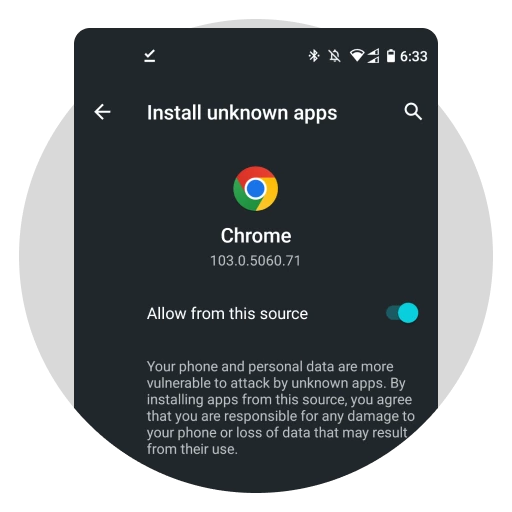This screenshot features a user interface on a white background. Central to the image is a gray circle enclosing the screen of a cell phone. At the upper right corner of the cell phone screen, icons for Wi-Fi, reception, battery charge, and the time, which reads 6:33, are displayed. Below this, in bold text, the phrase "Install unknown apps" is visible. An arrow pointing to the left and a magnifying glass icon to the right flank this text. In the central part of the screen, the round Google Chrome icon in its primary colors is displayed prominently, accompanied by the word "Chrome" in white text. Beneath the icon, the version number "103.0.5060.71" is listed. Further down, bold white text reads "Allow from this source," with a blue toggle button positioned to the right of the text, indicating the option to enable or disable the feature.